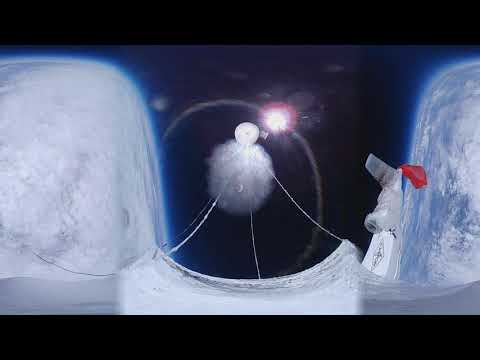The image appears to be a computer-generated depiction of outer space, set against a predominantly black or dark blue background. It is vertically rectangular and framed by horizontal black stripes at the top and bottom. Central to the composition is a pair of curved, grayish-white blocks that anchor the left and right sides of the frame, resembling abstract landscapes or structures with a bluish afterglow. Between these blocks is a wavy, gray formation that becomes more pronounced towards the center, curving downward seamlessly.

Extending outward from this central wave are thin gray strings connecting to a small, white-gray circular cloud, topped by a smaller, more defined grayish-white circle, akin to a simplified moon. Surrounding this dual-circle formation is a large, light gray halo, contributing to the ethereal quality of the scene.

On the right side of this halo, a bright, round object with a red halo—possibly representing a sun or another celestial body—adds a stark contrast. Additionally, a few faint white lines form a thin curved circle around the duo of circles, enhancing the sense of cosmic depth. The image includes unique features like variously colored ovals and a small red element, hinting at machinery or a flag, further suggestive of a space station or spacecraft setting.